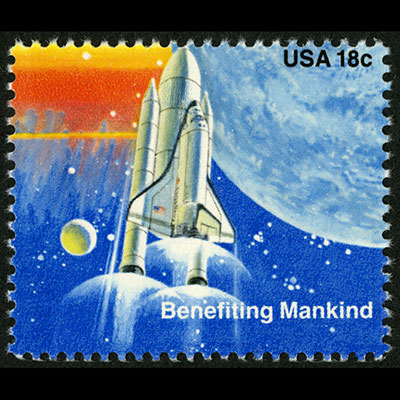This image depicts a vintage U.S. 18-cent postage stamp that illustrates a space shuttle, resembling the Challenger, on its booster rocket, shooting into space. The space shuttle is traveling upward, depicted with white lines and curves signifying speed and thrusters' effect. The illustration appears hand-painted.

The background of the stamp is predominantly blue at the bottom, dotted with white stars, and transitions to a reddish-orange at the top, implying a sunset or atmospheric glow. In the upper right, the moon or a planet, possibly Earth with its blue hue and white clouds, is visible. Additional planets and celestial objects can be seen, enhancing the cosmic scene.

The stamp bears the text "USA" and "18 C" in black font in the top right corner, and at the bottom right, the white text "benefiting mankind" is displayed. The stamp itself is bordered by perforated edges and placed on a black table with a black background.